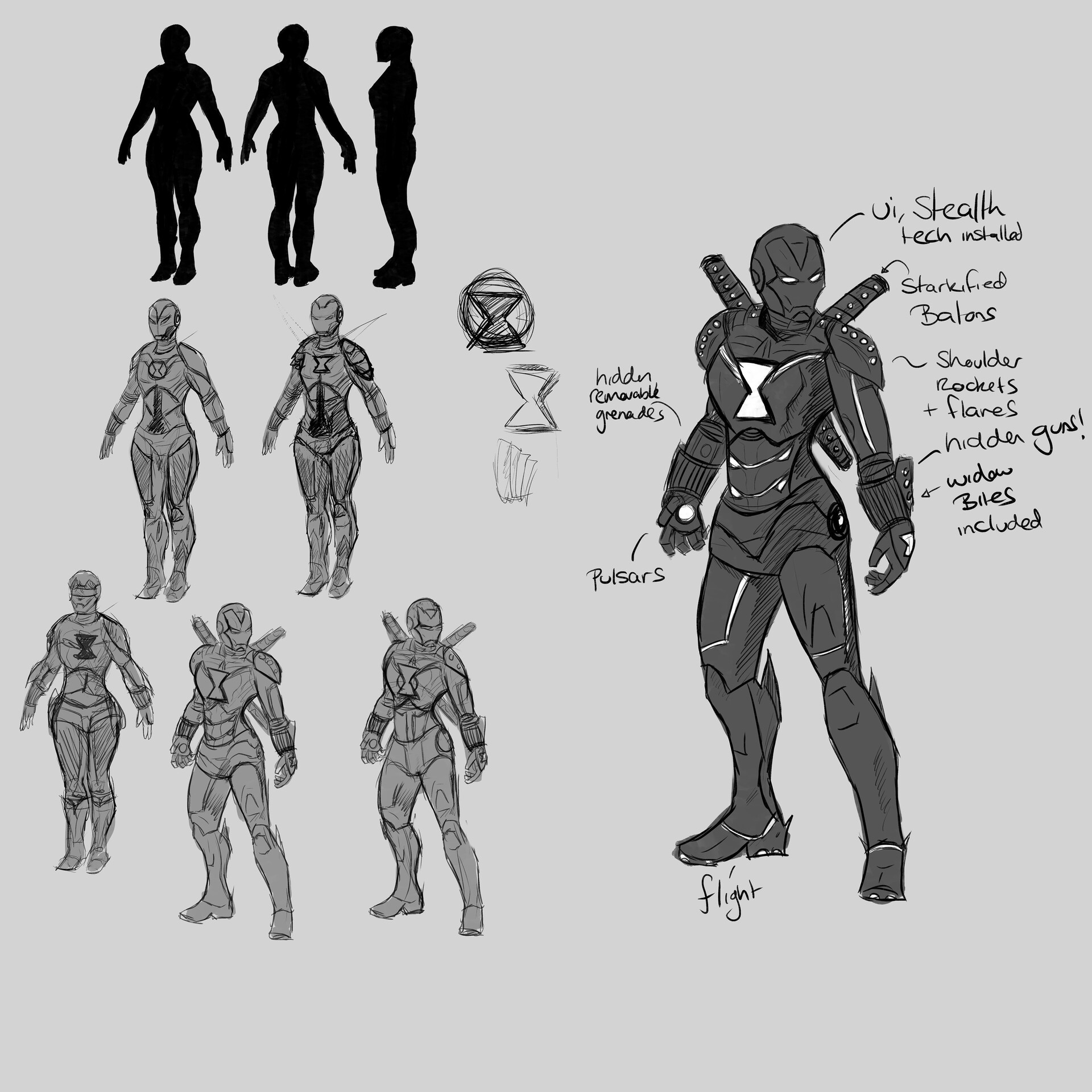This highly detailed black and white sketch depicts a female superhero character wearing a sleek, technologically advanced suit reminiscent of Iron Man from the Marvel Universe. The suit, illustrated head to toe, features a prominent Black Widow logo on the chest. The background of the image is gray, with the left side showing various stages of the character's development—from a basic black silhouette to detailed renderings of the suit from multiple angles, including front, back, and side profiles.

Hand-drawn annotations on the right side of the image describe the character's sophisticated equipment and weaponry. These notes, written in cursive, include mentions of "UI stealth tech installed" on the helmet, "starkified batons" on the back, "shoulder rockets and flares," "hidden guns" on the wrists, "pulsars" on the hands, and "widow bites." Additionally, details such as "removable grenades" and flight capabilities are indicated around various parts of the suit. This comprehensive artwork showcases the intricate design and functionality of the superhero's battle-ready uniform.